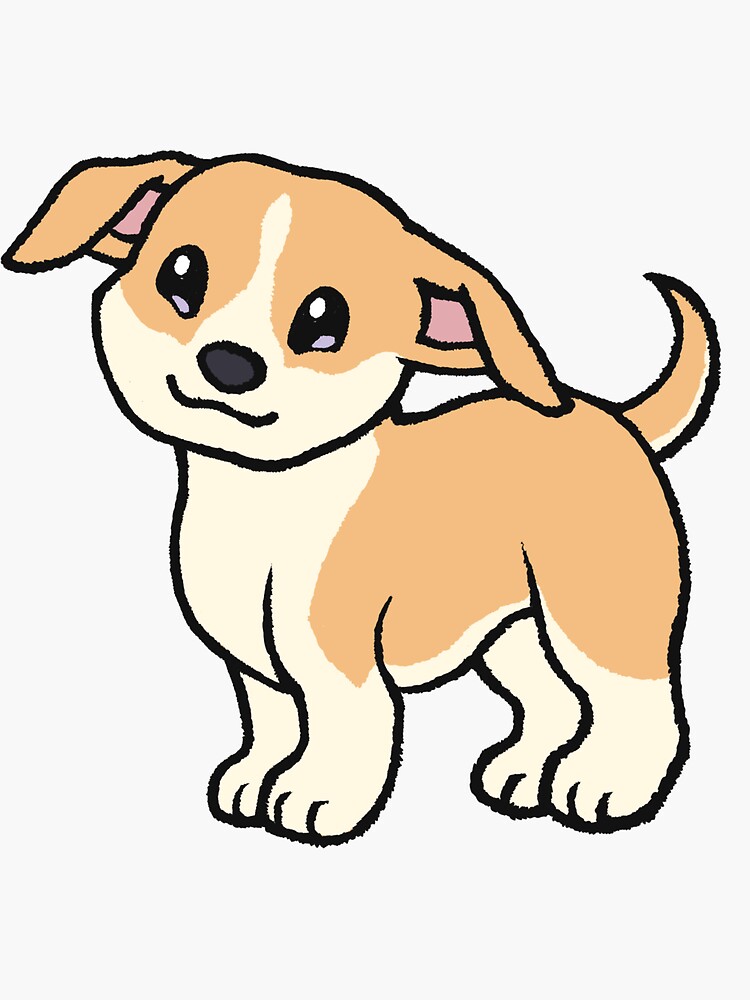This image is a detailed clip art depiction of a puppy, drawn electronically in a cartoonish style. The puppy stands upright, facing the viewer against a light gray backdrop. It is mostly cream-colored with a tan or orangish-brown pattern along its back, ears, and part of its tail. The dog's legs, chest, and around its mouth are cream-colored. Its ears, which are floppy, also show pink tufts peeking out from the bottom. The puppy's eyes are large and animated, featuring details of white and purple specks. It has a black, velvety nose and a charming, squiggly smile. The tail is short and appears to be wagging slightly, adding to the puppy's lively and cheerful demeanor. Overall, it's a cute and simple cartoon representation.